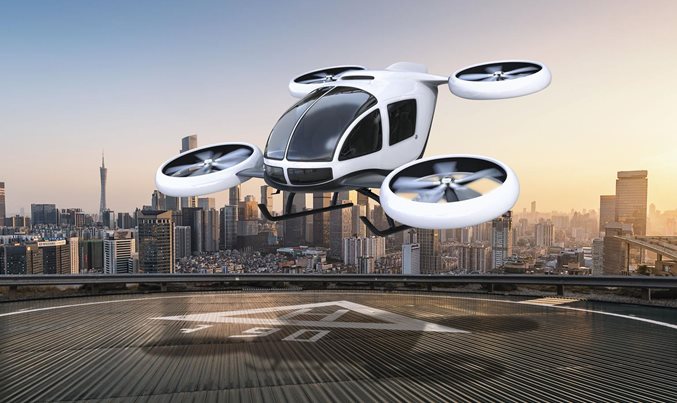This detailed, futuristic rendering showcases a sleek, modern helicopter, potentially a prototype or early production model of an electric vertical takeoff and landing (eVTOL) vehicle. The helicopter, primarily white with black trim and a black windshield, features four upward-facing rotor blades, two positioned at the front and two at the back, suggesting an innovative design for urban air mobility. It hovers above a gray helipad marked with a prominent white "90" and a large "H," indicating its readiness for landing or takeoff. The city skyline in the background, comprising an array of tall buildings in shades of gray and brown, highlights the urban setting where such vehicles might be used for short commuting trips. The overall image blends elements of cutting-edge technology and urban landscape, emphasizing the futuristic yet imminent reality of advanced aerial transport.